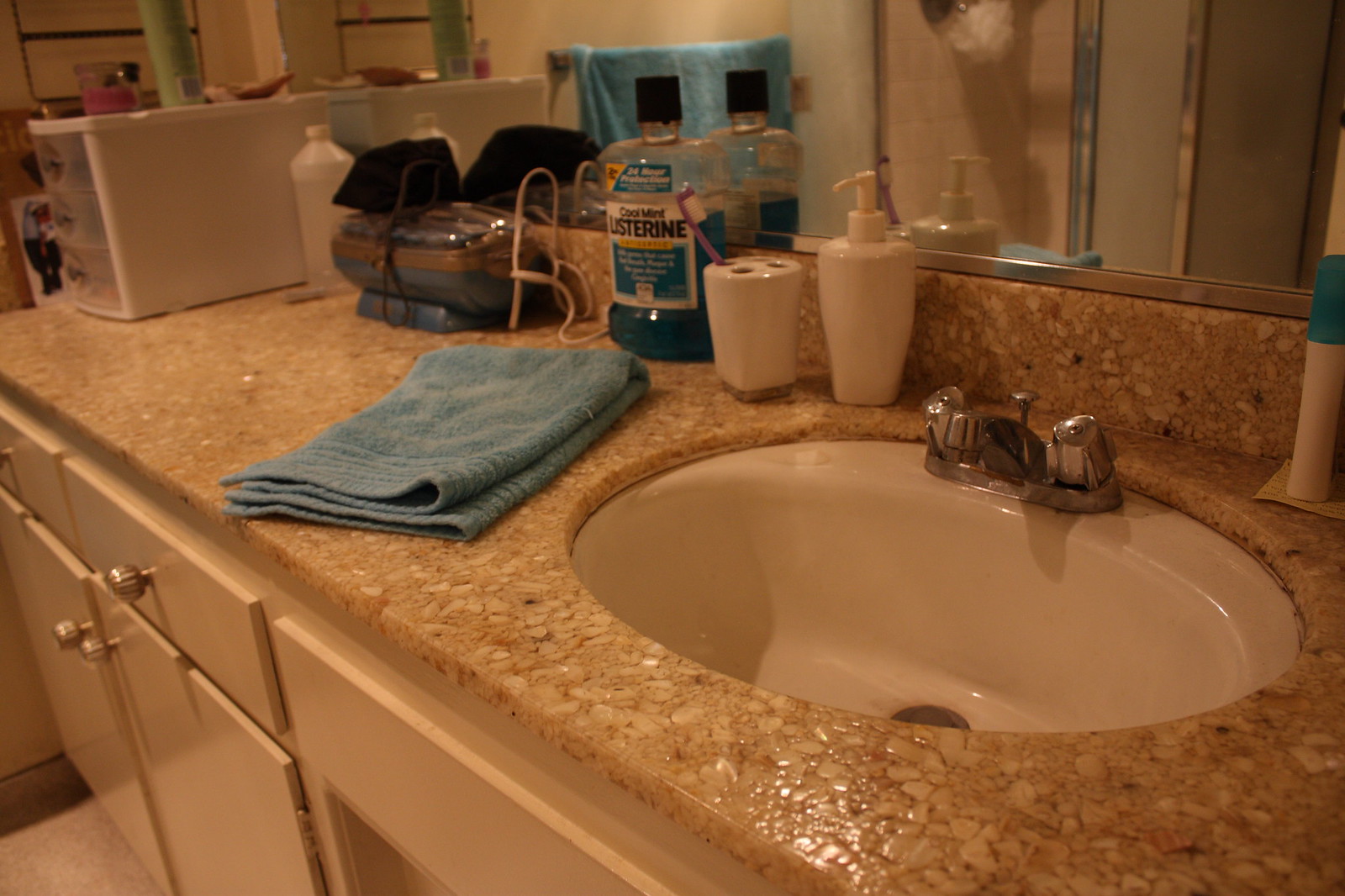This photograph showcases a well-organized bathroom countertop and sink area, captured from a slightly angled perspective originating from the bottom right corner. The white sink basin is accompanied by a sleek silver faucet with two handles for hot and cold water. The countertop, designed with a light brown and white pebble-like material, adds a touch of elegance to the space.

Above the sink hangs a mirror framed with a stylish silver border, reflecting the meticulous arrangement of bathroom essentials. To the left of the faucet sits a white soap dispenser with a pump top, positioned next to a toothbrush holder with four slots, one of which holds a solitary purple toothbrush.

Further left on the countertop is a neatly folded blue hand towel. Behind it stands a transparent blue bottle of Cool Mint Listerine mouthwash, prominently displaying the label. The cabinetry beneath the counter is cream-colored with glass handles and includes two drawers and two cabinets, offering ample storage.

Towards the far end of the countertop, a small three-drawer unit made of black or white plastic provides additional organization. The interplay of practical items and aesthetic choices makes this bathroom setting both functional and visually appealing.